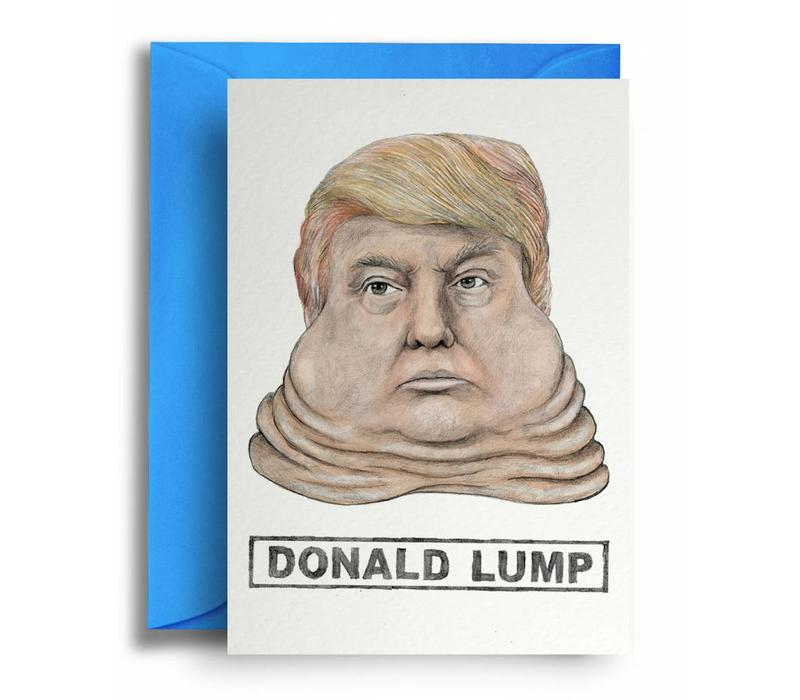The image showcases a color photograph of a greeting card, situated on top of a bright blue envelope against a completely white background, with shadows cast from the envelope. In the center of the white card, there is a detailed and well-drawn caricature of former President Donald Trump, emphasizing his distinctive features such as his combed-over blonde hair and a series of exaggerated, grumpy facial expressions with numerous fat rolls on his neck. The bottom of the card contains a black rectangular border with the humorous text "Donald Lump," suggesting a meme or a satirical take on the former president. The style of the image is political and likely designed for circulation on social media platforms.